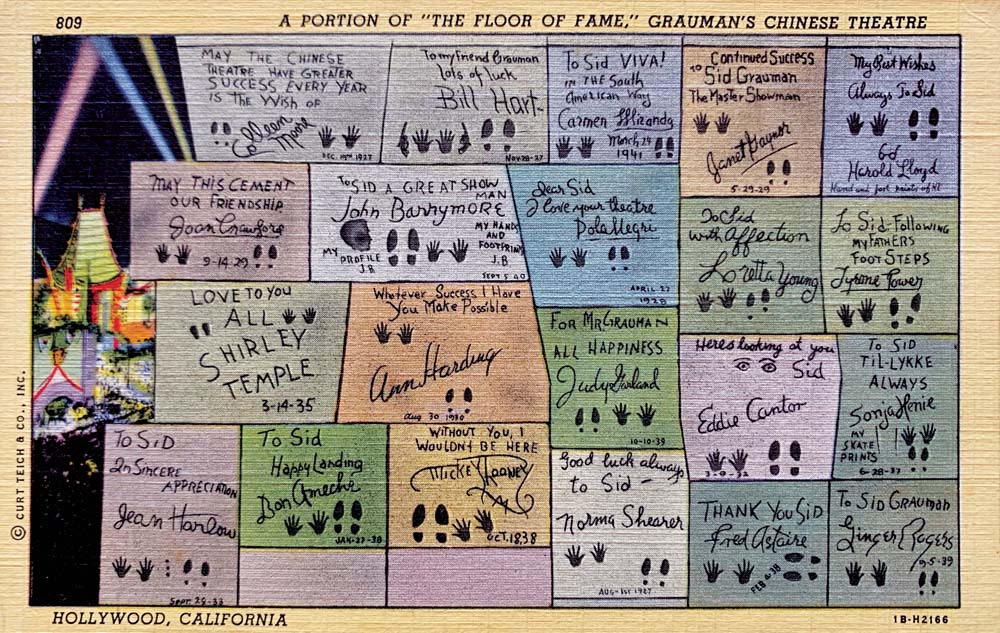The image features a detailed watercolor illustration of Grauman's Chinese Theater, renowned for its unique architectural style, characterized by a green roof, red walls, and colorful searchlights in lavender, blue, and yellow. The theater is framed by a tan rectangular background with a brown border, and prominently displayed at the top is the title, "A Portion of the Floor of Fame, Grauman's Chinese Theater." 

Below this title, there are roughly 20 rectangular tiles showcasing the handprints, footprints, and signatures of various celebrities, perpetuating their legacy in the cement. The detailed inscriptions capture heartfelt wishes to Sid Grauman, the theater's visionary, along with the hand and foot imprints of these illustrious figures.

Some of the noteworthy inscriptions include:
- Colleen Moore's 1927 wish: "May the Chinese Theater have greater success every year."
- Bill Hart's blessing: "To my friend Grauman, lots of luck," also dated 1927.
- Carmen Miranda's vibrant "To Sid Viva in the South American way," dated March 24, 1941.
- Janet Gaynor's tribute from 1929 and Joan Crawford's sentiment from 1929 as well.
- Harold Lloyd's undated message and John Barrymore's 1940 mark which includes his profile.

Additionally, the tiles document other stars like:
- Loretta Young, Tyrone Power, Shirley Temple (1935), and Anne Harding (noted as 1980 or 1930).
- Judy Garland's 1939 print, Eddie Cantor (1932), Sonia Henie (1937), Fred Astaire (1938), Ginger Rogers (1939), and Jean Harlow (1933).

To the left, there is a detailed depiction of the theater's exterior, with spotlights beaming into the sky, enhancing the iconic facade of Grauman's Chinese Theater. The bottom of the image acknowledges the copyright holder, Curt Teich & Company Incorporated, with "Hollywood, California" inscribed, indicating the prestigious location of this celebrated landmark.